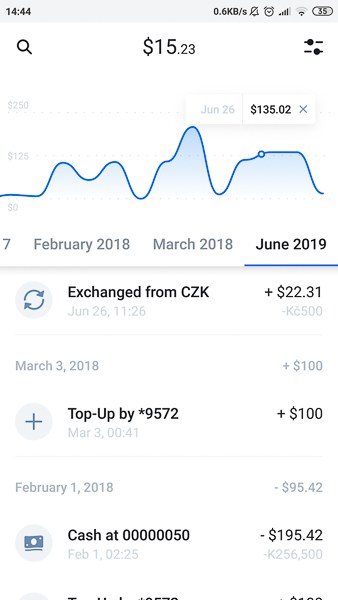This screenshot captures detailed stock information on a mobile device interface. Set against a gray background, the top-left corner displays the current time, 14:44. In the top-right corner, also on a gray background, various status icons are present: data usage at 0.6 kilobytes per second, a "Do Not Disturb" icon, an alarm bell icon, signal reception bars, a Wi-Fi signal indicator, and the number 35 within an oval.

Dominating the main section of the screenshot is a white background with black text. At the very top, there's a magnifying glass icon, likely for search functionality. Centrally, a bold figure of $15.23 is displayed, indicating the stock price, with a filter button situated to its right.

Beneath this, a dynamic line graph is featured, charting the stock's performance with a blue line that fluctuates, creating peaks and troughs, filled with a gradient blue color below the line. The left axis of the graph is scaled from $0 to $250, with a notable data point highlighted in a pop-up box reading "June 26th at $135.02."

Further below, three selectable date options are visible, allowing users to view stock data from specific periods: February 2018, March 2018, and June 2019.